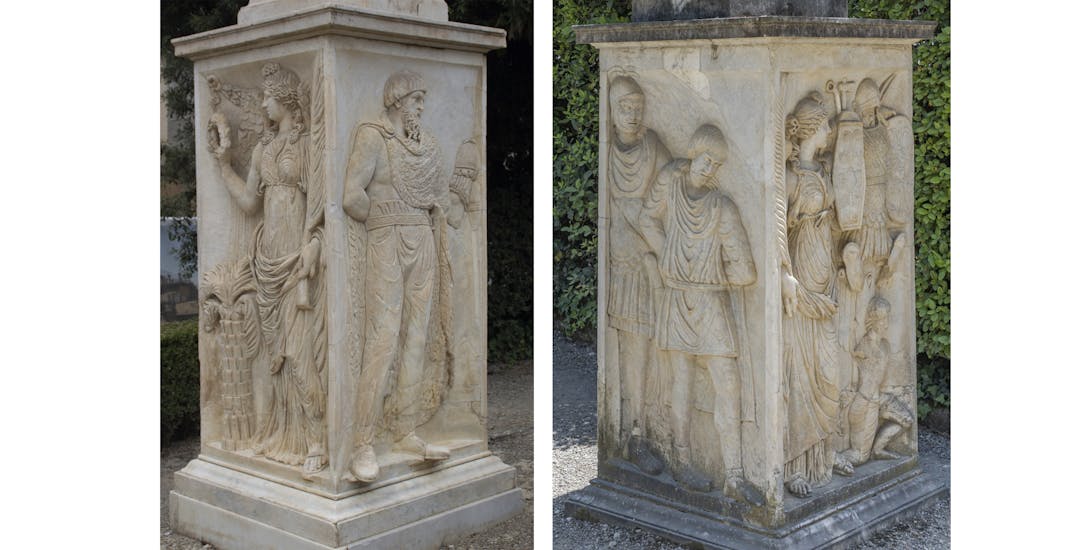This image is a collage of two side-by-side, color photographs, each capturing different sides of a pedestal base of what appears to be a classical-style Roman or Greek column or statue. The composition is split by a white line, and both images showcase intricate carvings that depict various figures in a classical relief style.

In the left photograph, the square-shaped pedestal is flanked by trees and paved ground in the background. The two visible sides feature etchings of people in classical attire with flowing robes. On one face, a lady is draped in a traditional dress, and next to her, a man in similar attire stands. The right photograph similarly shows two faces of what seems to be the same or a similar pedestal. On one side, there are detailed engravings of a man and a younger male figure, both adorned in flowing, simple robes. The adjacent side displays a woman with her hair pulled back and a small child crouched at her feet, next to another figure.

Both images are shot at an angle, capturing the vertices of the rectangular prisms and emphasizing the detailed craftsmanship of the classical carvings, which evoke an ancient Greek or Roman aesthetic. The carvings are primarily in beige and gray tones, suggesting a stone or ceramic material.